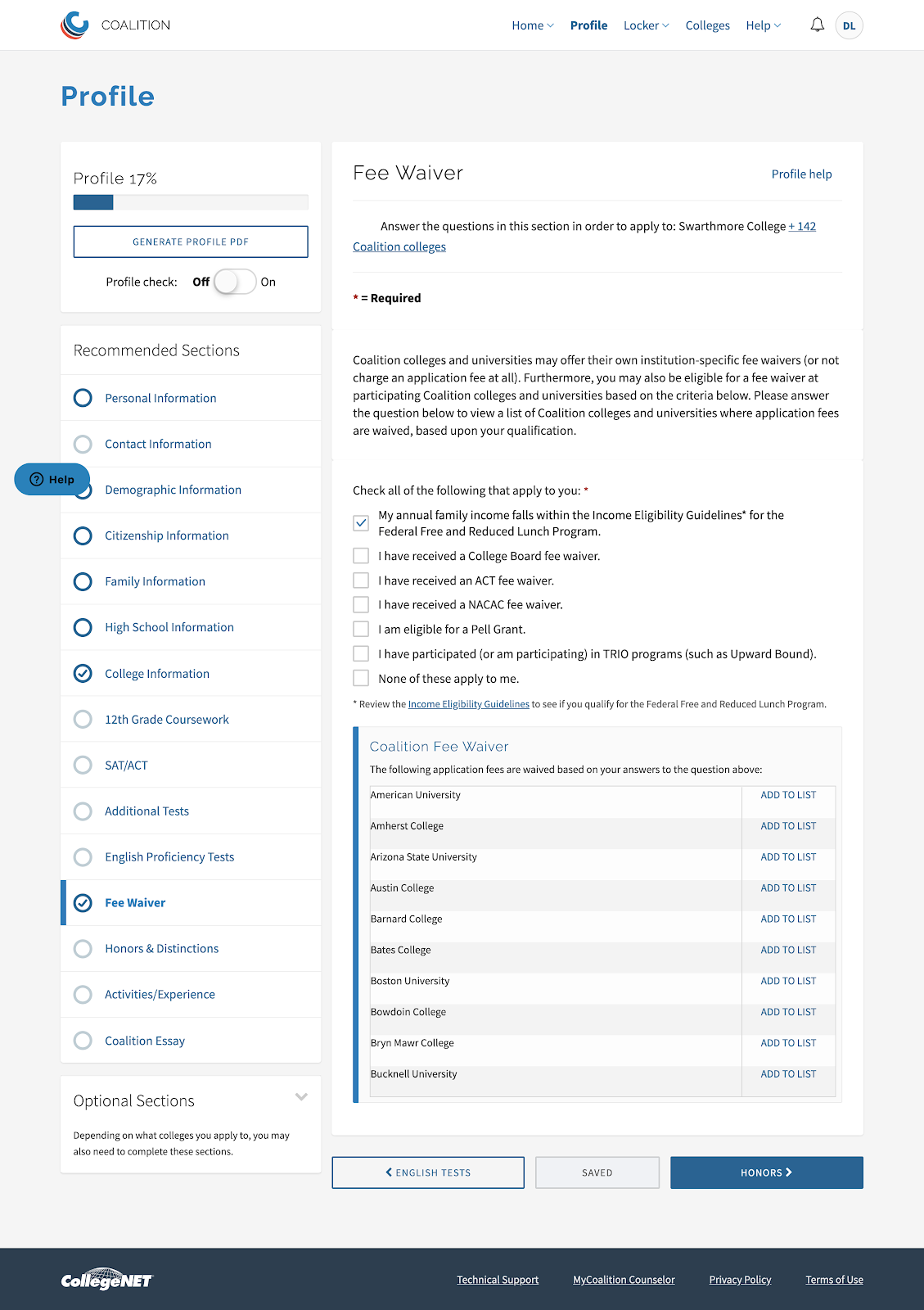The image is a detailed screenshot of a profile page on a website, indicated by navigation options such as "Home," "Profile," "Colleges," and "Help" displayed at the top. The "Profile" tab is visibly selected as it's bold, while the others are not. In the top left corner, the company name "Coalition" is shown with a stylized "C" logo.

Beneath the navigation bar, the word "Profile" is prominently displayed in bold blue text. There are several white text boxes below it. The first small rectangle shows "Profile 17%" indicating the completion percentage of the profile. A button below, assumed to say "Complete," and a toggle switch labeled "Profile Check" currently set to off, are also visible.

Further down, a longer vertical white text box labeled "Recommended Sections" contains approximately 18 radio buttons corresponding to different sections, such as "Family Information," "Contact Info," among others.

On the right side of the page, a white box resembles a sheet of paper with headings like "Fee Waiver" and "Profile Help." To the right of "Fee Waiver," a small blue-labeled white button reads "Profile Help." There's guidance text instructing users to answer questions in this section to apply for a specific college, possibly Swarthmore, though the text is very small. Below this, there's a checklist of criteria, with about seven or eight checkboxes. The top box, which is checked, pertains to annual family income.

Towards the bottom, there's a section labeled "Coalition Fee Waiver" with visually alternating white and blue bars, similar to a checkbook register, easing the distinction between different rows. At the very bottom, a black bar displays "CollegeNET" (with "NET" in capitals), and four items are listed to the right of this.